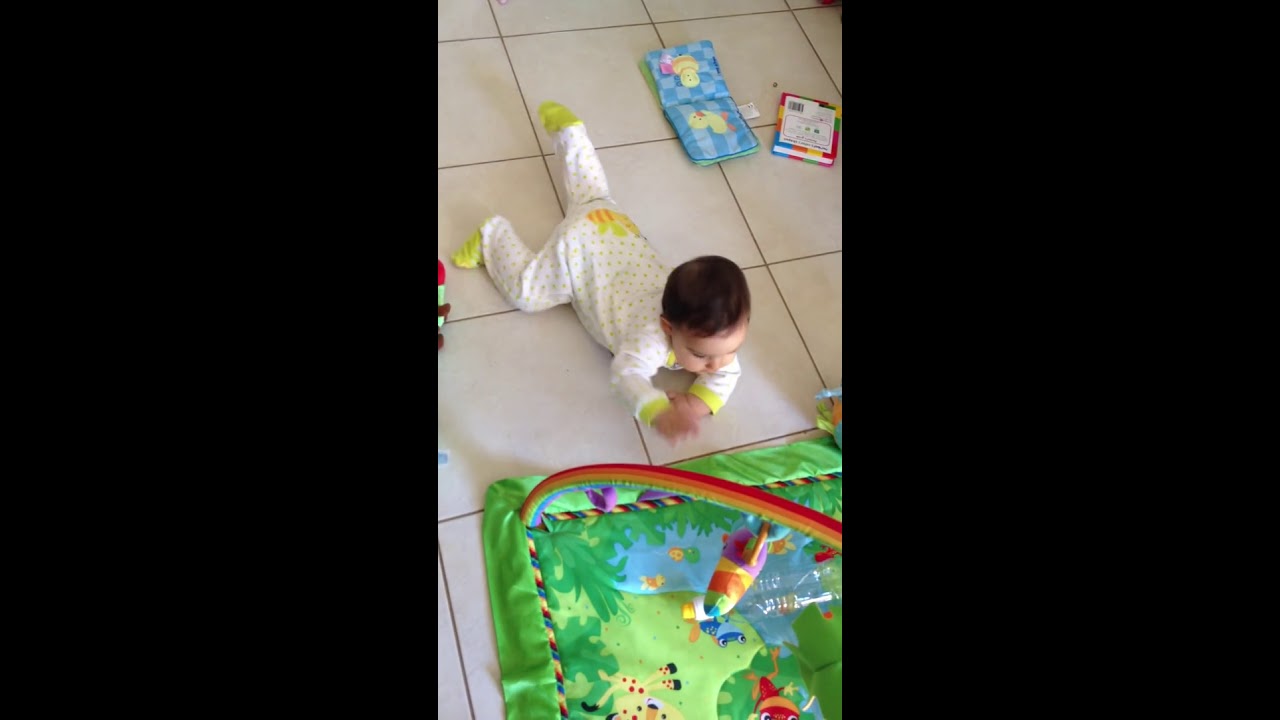This is a horizontal rectangular image with wide black bands on both sides, framing a narrow central photograph of a baby. The baby, with dark hair, is wearing a white onesie featuring yellow trim on the sleeves, feet, and possibly on the backside. He is laying on a white tile floor, surrounded by books with colorful covers. One book near his foot is blue with yellow butterflies, and another beside it appears to be open, displaying a picture of a duck. A third book, partially visible, is near his other foot. The baby has his hands folded in front of him and seems to be staring into a green playmat area in front of him, which features a variety of toys suspended from a semi-circular arch. The playmat itself is decorated with images of plants, animals like giraffes, and a sky backdrop. A rainbow figurine hangs from the arch, adding to the vibrant play environment. The baby seems happy and curious, possibly crawling towards the engaging play area.